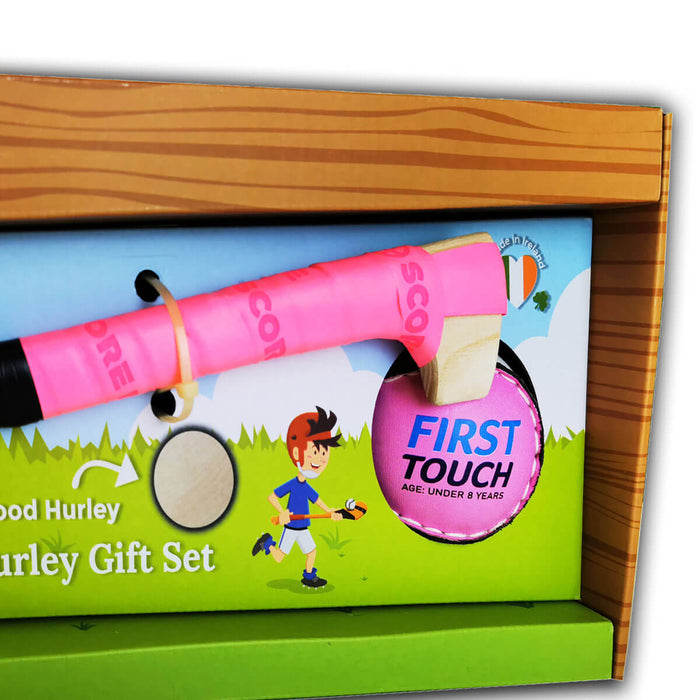The photograph showcases a toy, specifically a children's Hurley set still in its packaging. The toy comprises a lacrosse-like stick with a soft pink grip wrapped around the handle and a bare wooden tip. The set includes a ball with pink stitching, which prominently reads "First Touch, Age Under Eight Years." The packaging is made of cardboard with a woodgrain print on the outer edges, simulating a wooden appearance, while the central part features a graphic of grass and a child running through it, holding a cartoon version of the toy. The child wears a red helmet and demonstrates the toy in action. The toy is secured in its package with white zip ties, and to the left of the packaging, it reads "Good Hurley Hurley Gift Set." The overall scene depicts a bright, sunny day, indicating the toy is intended for outdoor play and introduces young children to the sport of lacrosse.